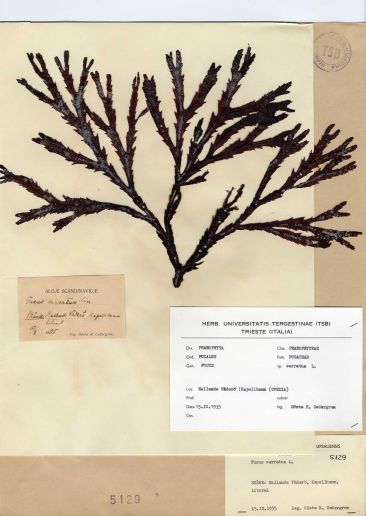The image depicts a piece of light tan paper, possibly pasted onto a brown cardboard or envelope-like surface, featuring a black, twig-like drawing of a plant or tree with numerous branches. Positioned at the top right of this paper is a stamp marked '753', and at the bottom right is another stamp that appears to read '5129'. Below the plant drawing are three small, rectangular pieces of paper. On the left side, there is a darker tan card with illegible black writing. On the right side, a larger white card with barely discernible black typed text is mounted. At the bottom right, a third, tan-colored card with black lettering rests next to a darker beige band stamped with what looks like 'S132', although the text is too small to be certain. The overall layout suggests the plant might be a dried specimen, with accompanying identification or scientific information.